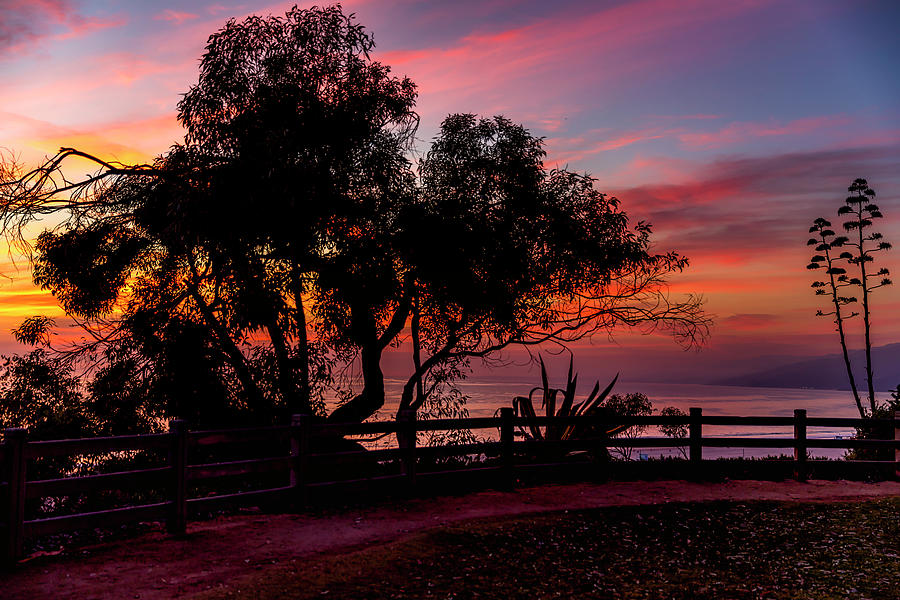This stunning outdoor photograph captures a serene evening sunset in a hilly or mountainous region. Dominating the horizon line, the setting sun paints the sky with striking hues of dark blues, vibrant pinks, warm yellows, and fiery oranges, blending into shades of lavender near the horizon. Wispy clouds stretch across the sky, reflecting the sun's rich colors. 

In the foreground, a curved walking path meanders through the scene, bordered by a wooden fence comprised of three horizontal slats interspersed with upright posts. The path, which could be brick or compacted dirt, leads past a small grassy area on the right, dotted with leaves.

To the left stands a tall, prominent tree, while thinner trees are dispersed in the distant background. Directly beneath the breathtaking sky, there is a tranquil lake nestled among the hills or mountains. The fence and trees cast dark silhouettes against the vivid sunset, with the path taking on a pinkish-purple tint from the fading sunlight.